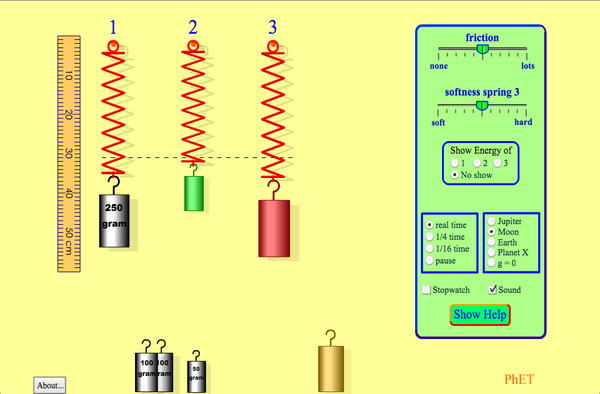The image depicts a rectangular graph artwork set against a light yellow, buttery background. On the left side, there is a dark yellow ruler with black markings at 10, 20, 40, and 50 centimeters. Adjacent to the ruler, three weights labeled in blue as "1," "2," and "3" are suspended by red zigzag lines. The first weight is a gray cylinder labeled "250 grams," the second is green, and the third is a larger red cylinder, each with hooks on top. Beneath these hanging weights, there is a collection of smaller silver weights, with one marked as "100 grams," another unreadable, and a third labeled "50 grams." A golden weight without a label is nearby.

To the right, a green rectangular box with a bright blue outline contains several charts and labels. The top bar reads "Friction," which spans a range from "None" to "A Lot." Below it, another bar labeled "Softness Spring" ranges from "Soft" to "Hard." Further down, the box reads "Show Energy Of," with options 1, 2, and 3 listed, though only the "No Show" option is checked. Additional sections within the green rectangle include a "Real-Time" mark on the left and "Moon" on the right, followed by "Stop Watching Sound," which is marked. At the bottom, there's a "Show Help" button, and in the lower right-hand corner, the letters "P-H-E-T" appear in red print.